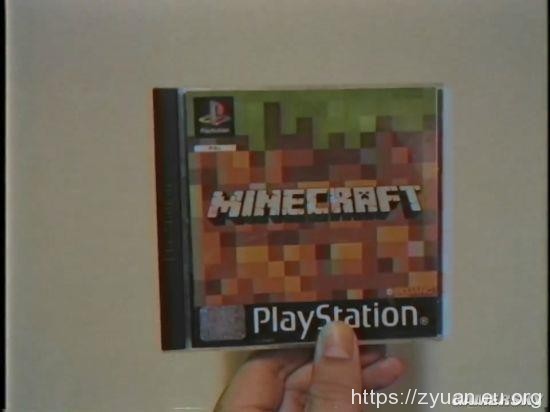The image depicts a left hand holding a Minecraft CD case. The hand is positioned centrally, with the thumb, index finger, middle finger, and ring finger visible, gripping the case. The CD case features the iconic pixelated aesthetic of Minecraft, with the game's title, "Minecraft," prominently displayed in the center. The casing has a primarily brown tone, with the top part rendered in green, suggesting a landscape element typical of the game. In the upper left corner of the case, a PlayStation logo is visible, indicating the platform for which this version of the game is designed.